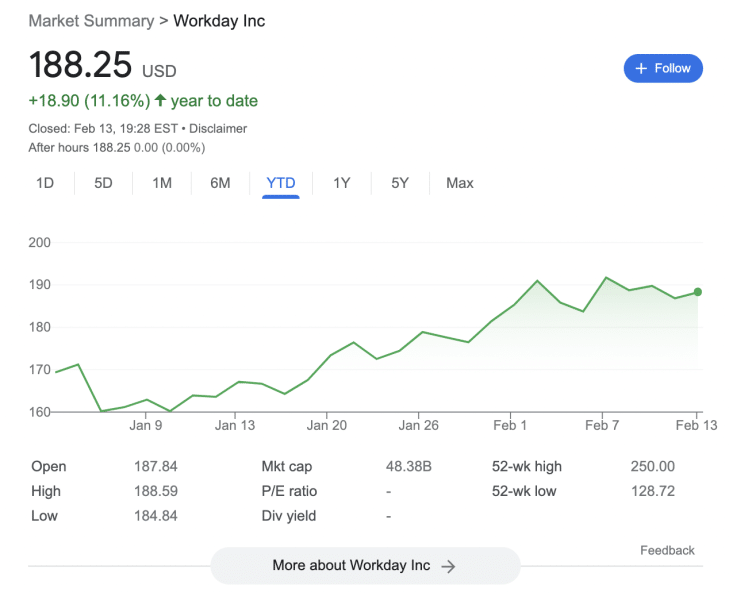The image portrays a detailed Market Summary page for Workday, Inc. At the top, the title "Market Summary > Workday, Inc." is prominently displayed. Below the title, the current stock price is shown as "188.25 USD" in black, with a gain of "+18.90 (11.16%)" highlighted in green, accompanied by an upward arrow indicating a positive year-to-date performance. 

The next line indicates the market status with "Closed Feb 13th, 19:28 EST" followed by a disclaimer. It also shows the after-hours stock price, listed as "188.25" with no change, as denoted by "0.00 (0.00%)."

There is a graph depicting the stock's performance over various time intervals ranging from "1D, 5D, 1M, 6M, YTD" (highlighted in blue) to "1Y, 5Y, and Max." The vertical axis of the graph spans from 160 to 200, while the horizontal axis is marked with dates: "January 9th, January 13th, January 20th, January 26th, February 1st, February 7th, and February 13th."

Also included are key statistics in tabular form:
- Open: 187.84
- High: 188.59
- Low: 184.84

Additional statistics include:
- Market Cap: 48.38B
- P/E Ratio: --
- Div Yield: --

Furthermore, the 52-week high and low are listed as:
- High: 250.00
- Low: 128.72

At the bottom of the page, there is an option "More about Workday Inc." accompanied by an arrow, and a gray area designated for "Feedback."